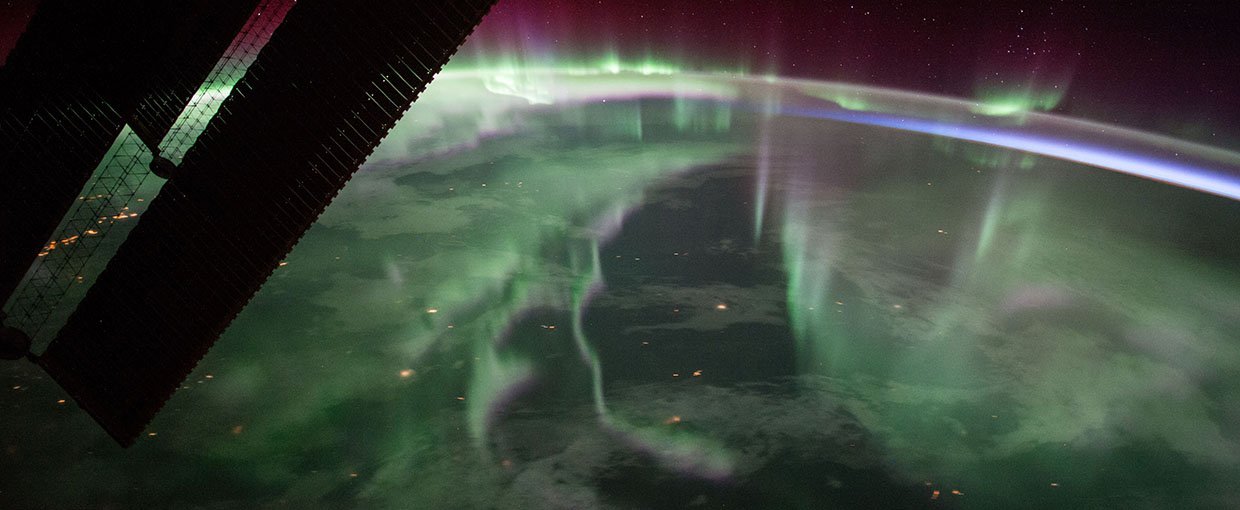The image depicts a night scene with a dark, black background, possibly taken from space using special photography or from a satellite. The setting appears to be above Earth, capturing an aurora borealis event with ethereal green and purple lights emanating from the planet's surface into the sky. The green lights are especially bright, casting a warm glow and creating shades of green and lavender in the atmosphere. Along the left side of the image, a rectangular black structure with a rigid bottom, which resembles a satellite or a metal fan commonly used in barber shops, can be seen. The overall scene is filled with muted yet vivid colors, depicting a surreal and mesmerizing view of the Earth's atmosphere blending with the vast, star-studded darkness of space.